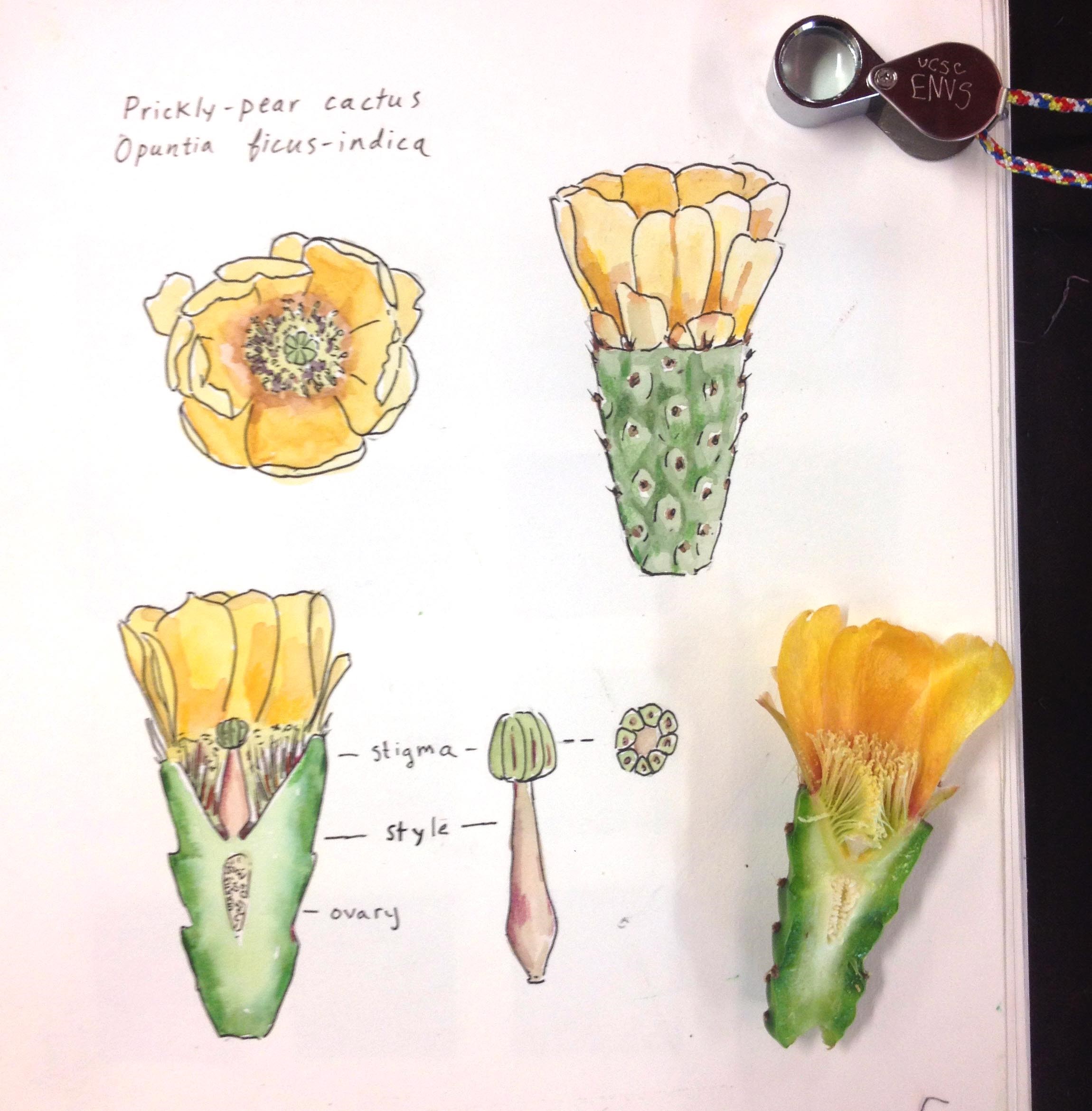This image is a detailed anatomical illustration of a prickly pear cactus (Opuntia ficus-indica), hand-drawn on a white sheet of paper. The title "Prickly Pear Cactus" appears at the top in black, along with its Latin name, "Opuntia ficus-indica." The drawing features multiple perspectives: a top view displaying white and yellow petals, a side view showing the cactus resembling a pineapple with a flower, and a cross-sectional view revealing the internal structures such as the stigma, style, ovary, and seeds. The illustration also uses a variety of colors including yellow, green, white, black, gray, red, and blue. Additionally, the bottom right of the image includes a real cross-section of a prickly pear cactus for comparison, demonstrating the accuracy of the hand-drawn illustration.